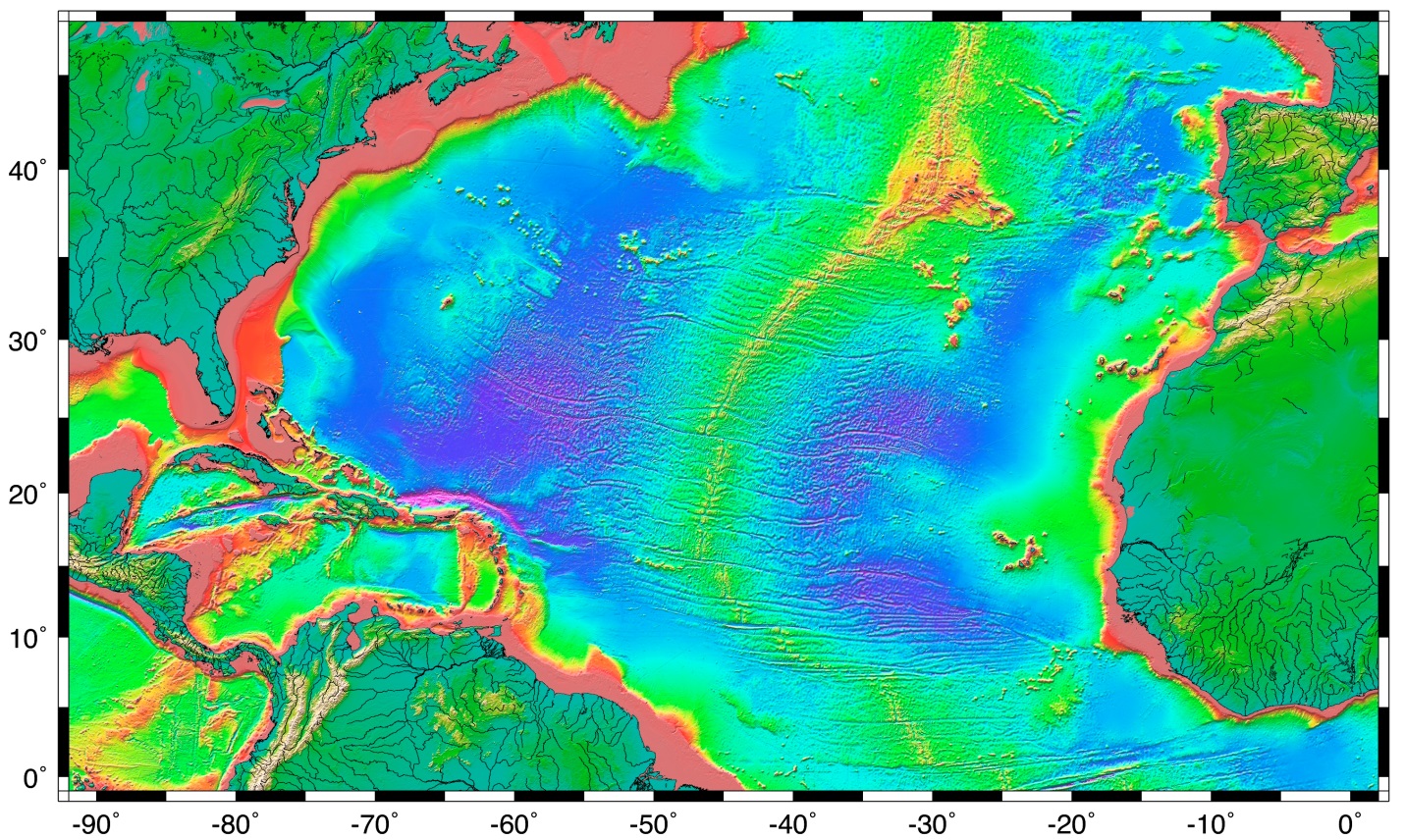This image features a vibrant and detailed map focusing on the Atlantic Ocean and surrounding continents. The map is bordered with black and white stripes and marked with a degree grid: vertically from 0 to 40 degrees and horizontally from 0 to -90 degrees. From the left side, North and South America are visible, while on the right side, it shows the western parts of Africa and the Iberian Peninsula. The primary emphasis is on the ocean, depicted in deep blue to represent water, with surrounding colors including green, yellow, red, and peach. These colors seem to indicate various data points, possibly related to water temperature or topographic features such as underwater mountain ranges. The map lacks a legend, leaving it unclear whether the colors denote temperature gradients or other oceanographic measurements. Notable areas include a distinct red along the coasts and a prominent mountainous range in the ocean's center, highlighted in green and red.